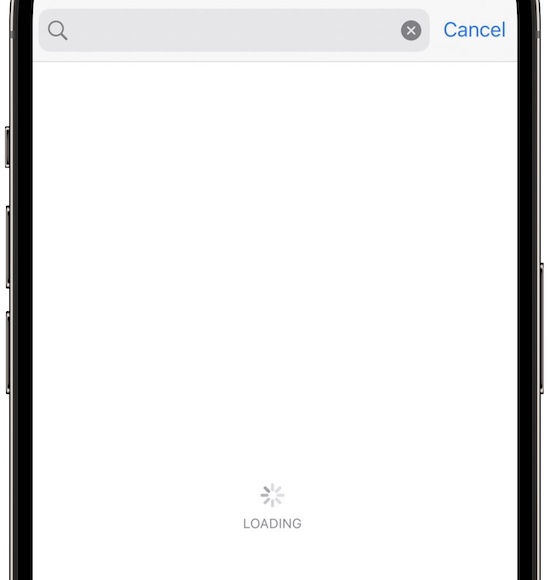This image is a cropped screenshot of a cell phone's screen that appears to be stuck on a failed loading page. The top and bottom portions of the phone are not visible in the image. The housing on both the left and right sides of the phone is a silver or white color. On the left side, three vertical buttons protrude from the housing, while on the right side, there is a single, longer vertical button located towards the center.

The upper part of the screen displays a gray background with an oval search bar. The search bar includes a magnifying glass icon on the left and a dark gray circle with a gray "X" inside of it on the right. Bold blue text reading "Cancel" is positioned on the far right. Directly below this is a thin, pale gray line.

The central area of the screen is an off-white, bare background. At the bottom, there is a circular loading icon resembling the petals of a flower with lines at the clock positions of 12, 2, 3, 4, 6, 7, 9, and 11 o'clock. Below this icon, the word "loading" appears in gray lettering.